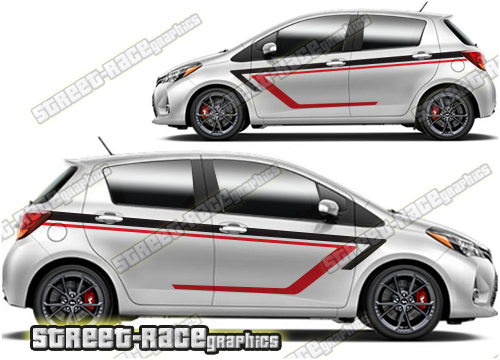The image depicts a silver, four-door economy car with black wheels, showcased in two different views on a white background. The upper view features the car's nose pointing left, and the lower, larger view has the nose pointing right. Both side views reveal the car's sleek design with black and red racing stripes running along the sides, perfectly accentuating the vehicle's sporty allure. The red stripe traces a path below the black stripe, traveling horizontally, down, and then back to the left. The graphic text "Street Race Graphics" is prominently displayed across the image at various angles, resembling a watermark, and is also bolded in gray with a black border at the very bottom. The compact appearance of the car, with a hatchback-like rear end, suggests practicality combined with a racing-inspired aesthetic.